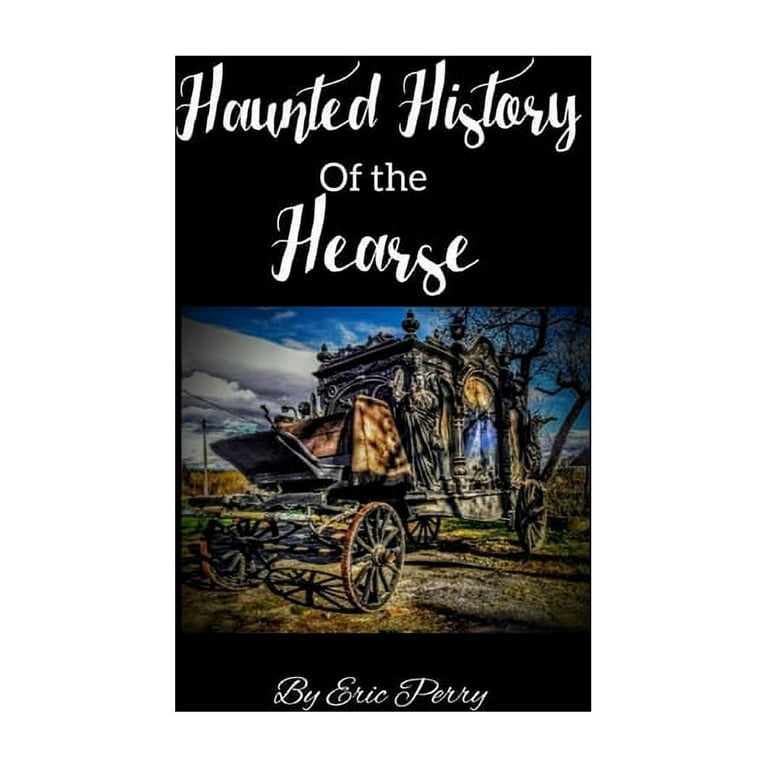This image depicts the cover of a book titled "Haunted History of the Hearse," written by Eric Perry. The book cover is predominantly black, featuring a color photo in the middle portion. The title, in white text, is presented in a gothic calligraphic font, with "of the" in a serif font style.

The central image showcases an ornate, old-fashioned, horse-drawn hearse that resembles a miniature mausoleum or a small administrative building. The hearse, from the 19th century, is crafted from dark wood, giving it a macabre and morose appearance. It is adorned with intricate carvings, including statues and ornate columns, and has a gothic church-like design with arched glass windows on the side, revealing a casket within.

The hearse is stationed on a grassy area, backed by a clear blue sky dotted with white, puffy clouds and a tree. The front area features a wooden bench where the undertaker would sit, and thin wooden wheels, emphasizing its antique design. The overall scene evokes a spooky, gothic ambiance that complements the theme of the book. The author's name, Eric Perry, is noted at the bottom of the cover in a white scripted font.